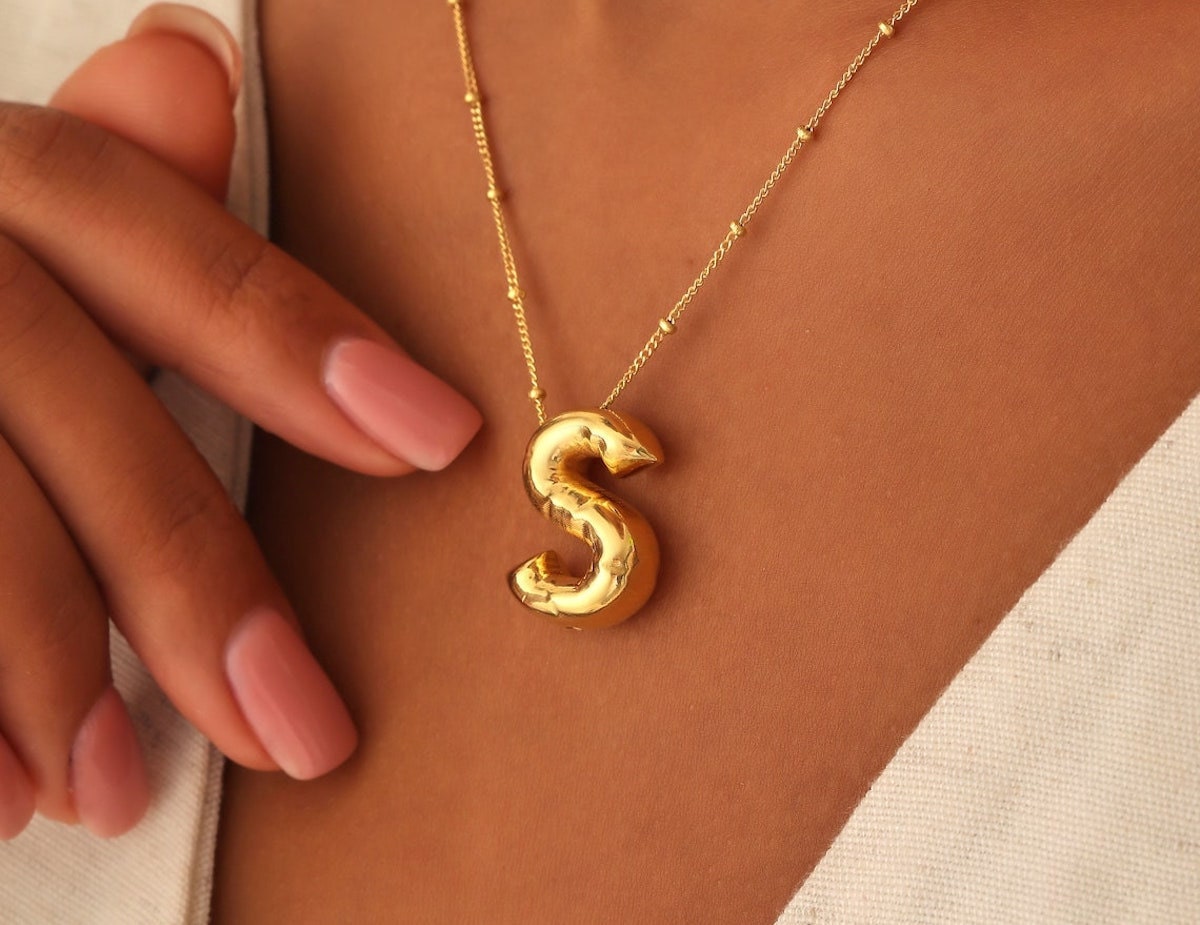The close-up photograph captures the chest of a tanned-skinned woman, showcasing her elegant gold necklace which features prominently with a large, bubble-letter 'S' pendant. The necklace is adorned with small gold spheres evenly spaced along the chain. She is wearing a white top with a deep V neckline. Her right hand, with well-manicured, light pale pink acrylic nails, is gently resting on her chest, her fingers subtly reaching towards the 'S' pendant. The visual emphasis is on the gold necklace and pendant, framed by her hand and neckline.